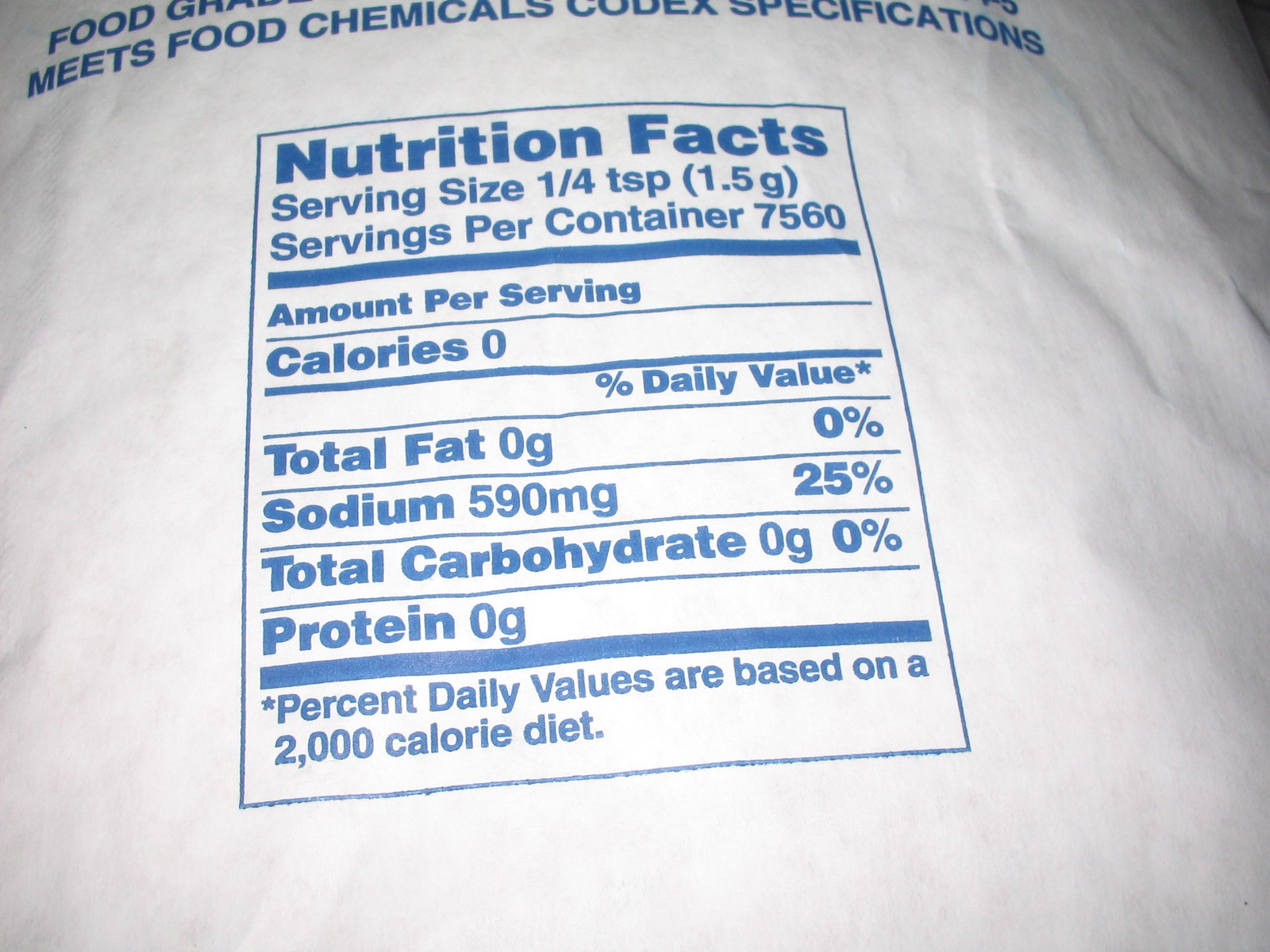This is a horizontal photograph showcasing the back of a white, curved food product sack, which resembles a bag of flour or rice. Prominently displayed in blue lettering at the top, we can partially see the word "Food," followed by the letters "G," "R," with the rest disappearing off the top edge of the image. Directly beneath this, a line informs us that the product meets the "Food Chemicals Codex specifications."

The lower portion of the sack features a detailed Nutrition Facts box also printed in blue. It meticulously lists the serving size as 1 1/4 teaspoons (1.5 grams) and indicates an astounding 7,560 servings per container. The nutritional breakdown per serving shows 0 calories, 0 grams of total fat, and 590 milligrams of sodium, which constitutes 25% of the recommended daily intake. Based on the high sodium content and suggested serving information, this is likely a photograph of a large container of salt.